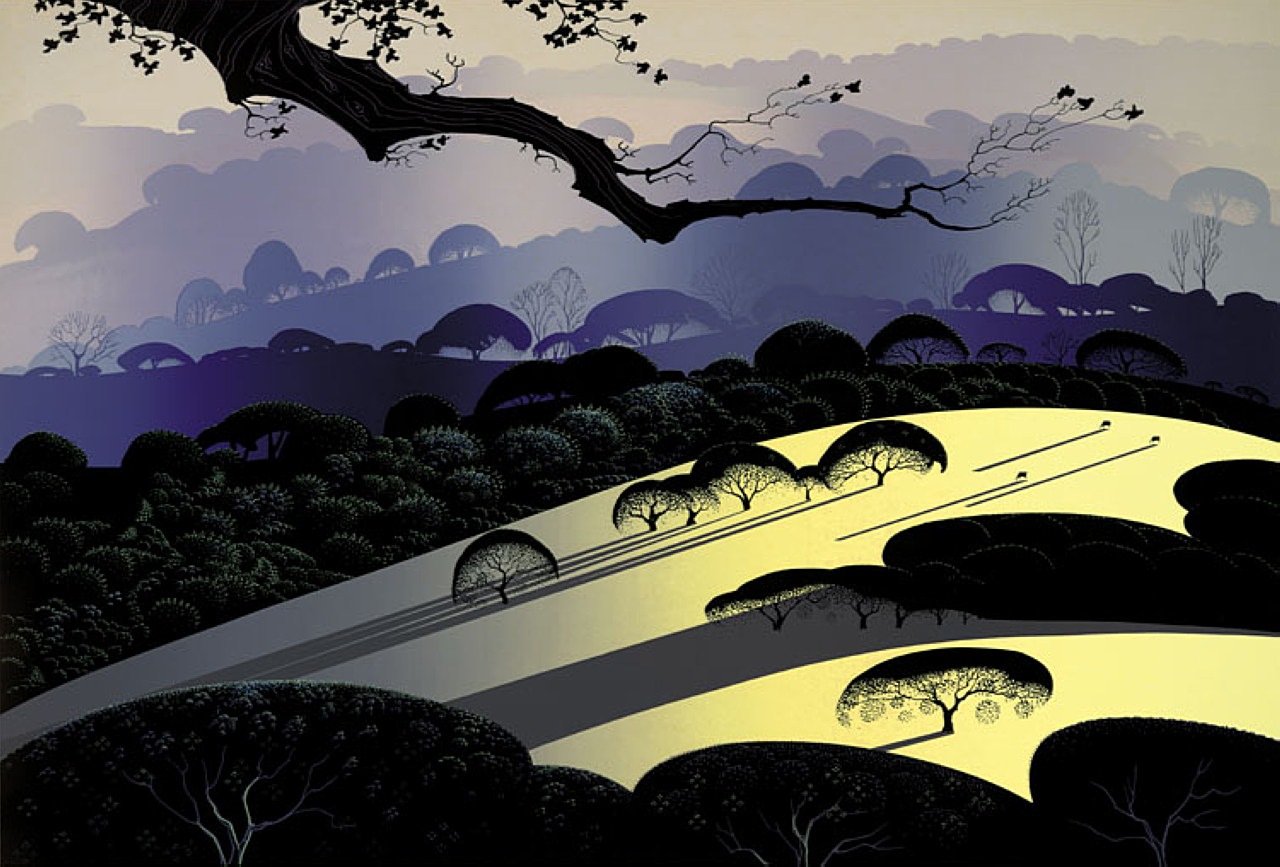The image is an intricate and detailed painting of a forest landscape at night, with hints of early dawn. A significant light source from the top left casts a white glow over portions of the scene. The dense and closely-packed trees are predominantly dark green, with some taller ones in the background that reveal more depth in the composition. The trunks of these trees are gray. Two prominent yellow rays of light cut through the otherwise foggy and dark environment; one arcs slightly from the bottom center to the center right, while the other takes a more vertical path from the bottom toward the center right. 

In the mid-ground, the forest density increases, and the trees begin to take on purple hues, creating silhouettes that appear slightly transparent against the backdrop. This atmospheric effect is accentuated by the fog aforementioned, enhancing the depth and mystique of the forest.

A notable feature is the surface in the foreground, which appears as a hill with a flat, yellow hue transitioning into a blue gradient toward the left, free from heavy vegetation. The shadows cast by the trees on this hill are long, suggesting the light source is far away. Near the top left corner, a large branch intrudes into the scene, adorned with smaller leaves, adding another layer of detail. The sky in the background is predominantly white, contrasting starkly with the darker hues of the forest, adding an ethereal quality to the painting.